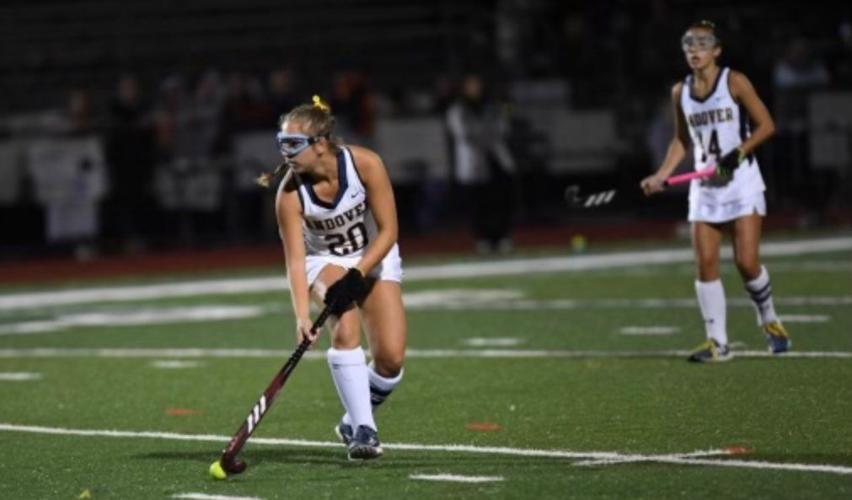In this nighttime outdoor photograph, two young women are playing field hockey on a green, well-marked field. Both are part of the Andover team, distinguishable by their white jerseys and shorts, paired with long white socks. The player in the foreground, wearing Andover number 20, has blonde hair tied back with a yellow ribbon and is focused away from the camera, possibly towards the goal. She sports a black glove on her right hand and black sneakers, and wears goggles while controlling a black and burgundy hockey stick next to a yellow ball on the ground. Behind her, number 14, who appears to be African-American, also wears a black glove on her right hand, and is holding a pink and black hockey stick with white stripes. She is looking towards the other player. The background is dimly lit, blurry, and populated with out-of-focus spectators, suggesting a setting at a well-attended night game.